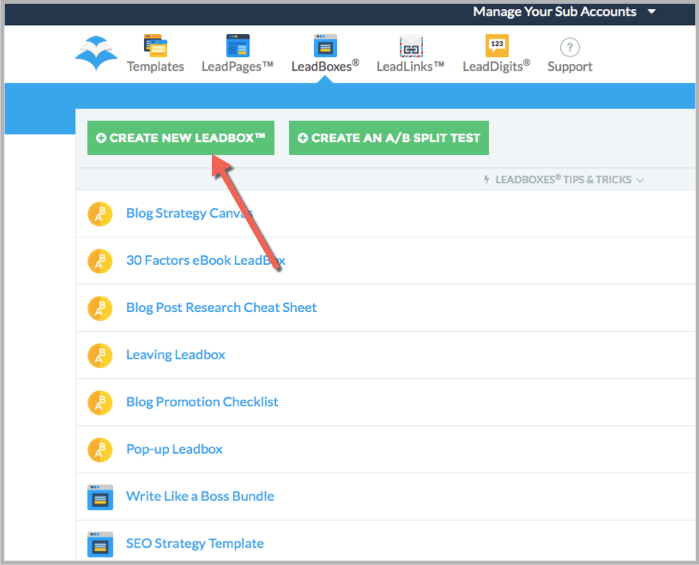Screenshot from the Leadboxes App: This screenshot showcases the interface of the Leadboxes app, highlighting an ongoing tutorial to create a new Leadbox. In the top right corner, there's an option labeled "Manage Your Subaccounts." The app provides a navigation menu at the top with various labels such as Templates, LeadPages, LeadLinks, LeadDigits, and Support. The selected section is indicated by the third icon, "Leadboxes." A prominent red arrow points to the "Create New Leadbox" button, emphasizing it as the next step, typical of a tutorial guide. Adjacent to this button is the "Create an A-B Split Test" option, allowing for split testing capabilities. Below these buttons are additional resources titled "Leadboxes Tips and Tricks," along with a list of items for selection which include Blog Strategy Canvas, 30 Factors Ebook Leadbox, Blog Post Research Cheat Sheet, Leaving Leadbox, Blog Promotion Checklist, Pop-Up Leadbox, Write Like a Boss Bundle, and SEO Strategy Template. The image serves as a detailed instructional guide for users navigating the Leadboxes app.